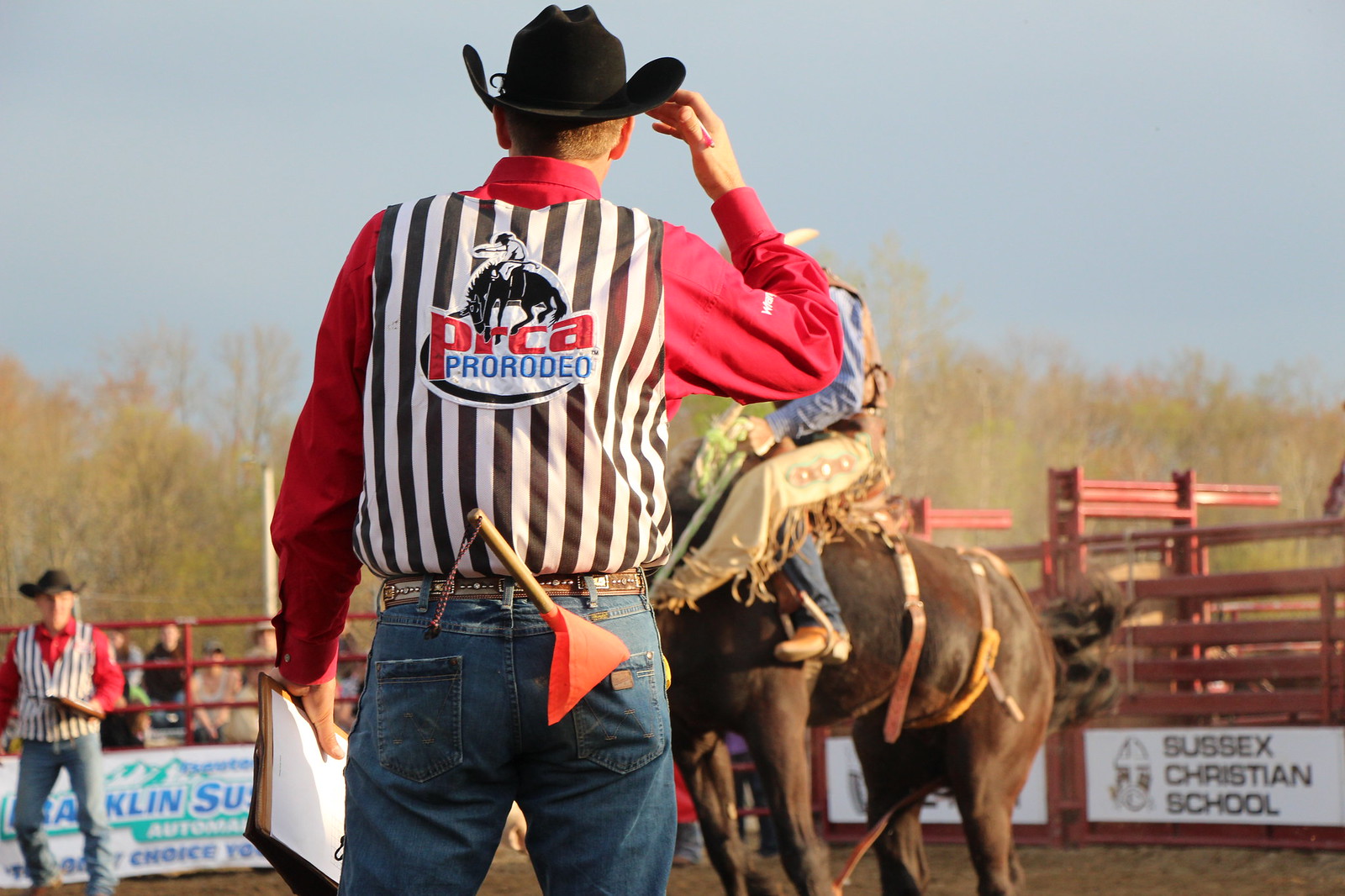The image depicts an outdoor rodeo event set against a smooth blue sky. Centrally positioned are two referees wearing black and white striped shirts with 'PRCA Pro Rodeo' emblazoned on the back. Each official dons a black cowboy hat, with the one in the center also sporting a red shirt underneath his vest, blue jeans, and holding an orange flag in his back pocket. Adjacent to the referees is a cowboy sitting atop a brown horse, clad in a brown vest, blue shirt, white cowboy hat, and chaps. 

To the side, ads and sponsors' banners line the perimeter of the arena, notably including one for Sussex Christian School. The fence encircling the rodeo grounds partially obscures some ads. In the background, leafless trees frame the scene. The detailed composition captures the dynamic atmosphere of the rodeo, highlighting both the participants and the surrounding environment.